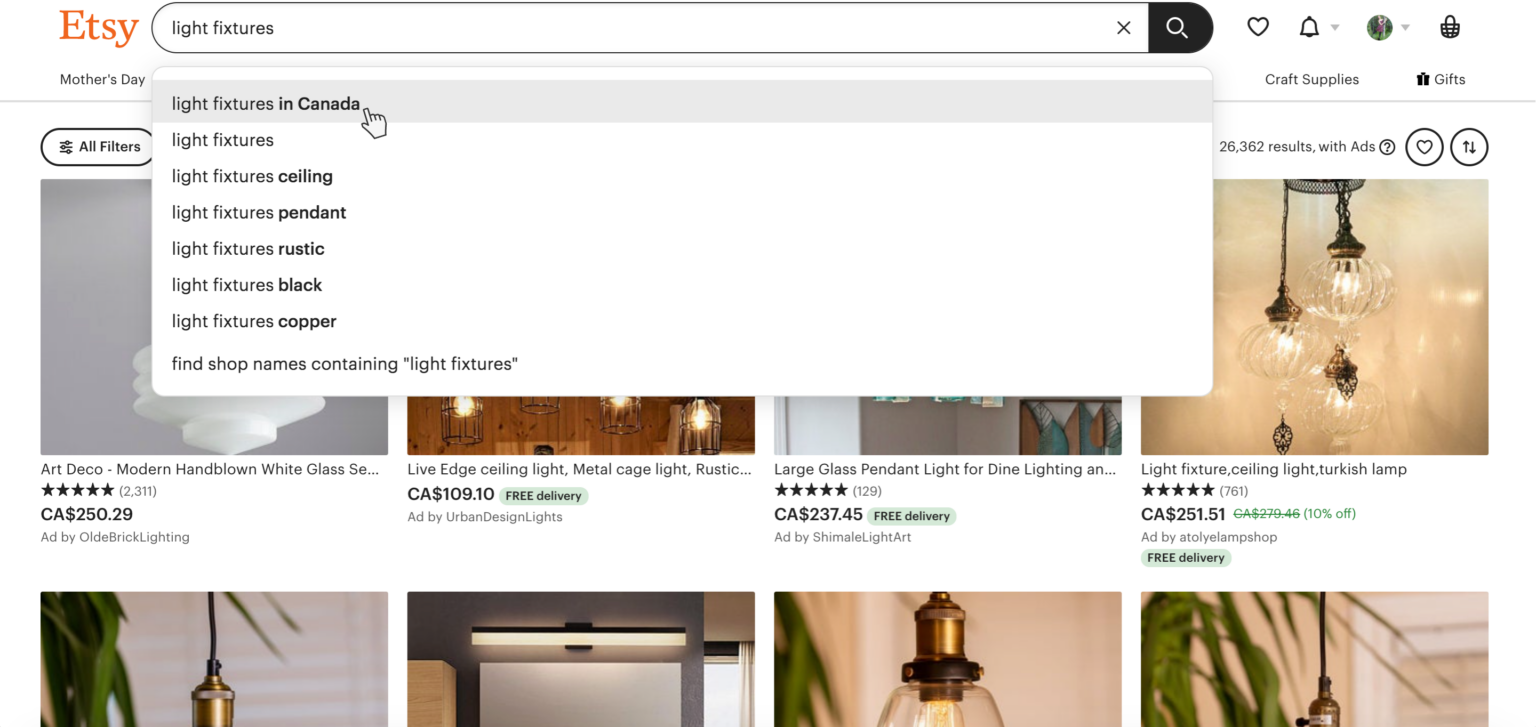This is a screenshot of an Etsy website page set against a solid white background. In the upper left corner, the Etsy logo is prominently displayed in bright orange text. To the right, a search bar contains the search query "light fixtures." Below the search bar, a white suggestion box lists related search terms such as "light fixtures in Canada," "light fixtures," "light fixtures ceiling," "light fixtures pendant," "light fixtures rustic," "light fixtures black," "light fixtures copper," and "find shop names containing light fixtures." 

Behind this, there are visible parts of eight search result images. The first item on the left features an Art Deco modern hand-blown white glass pendant light fixture. On the far right, there is a listing for a ceiling light fixture, specifically a Turkish lamp, which has garnered a five-star rating from 761 reviews and is priced at $251.51.